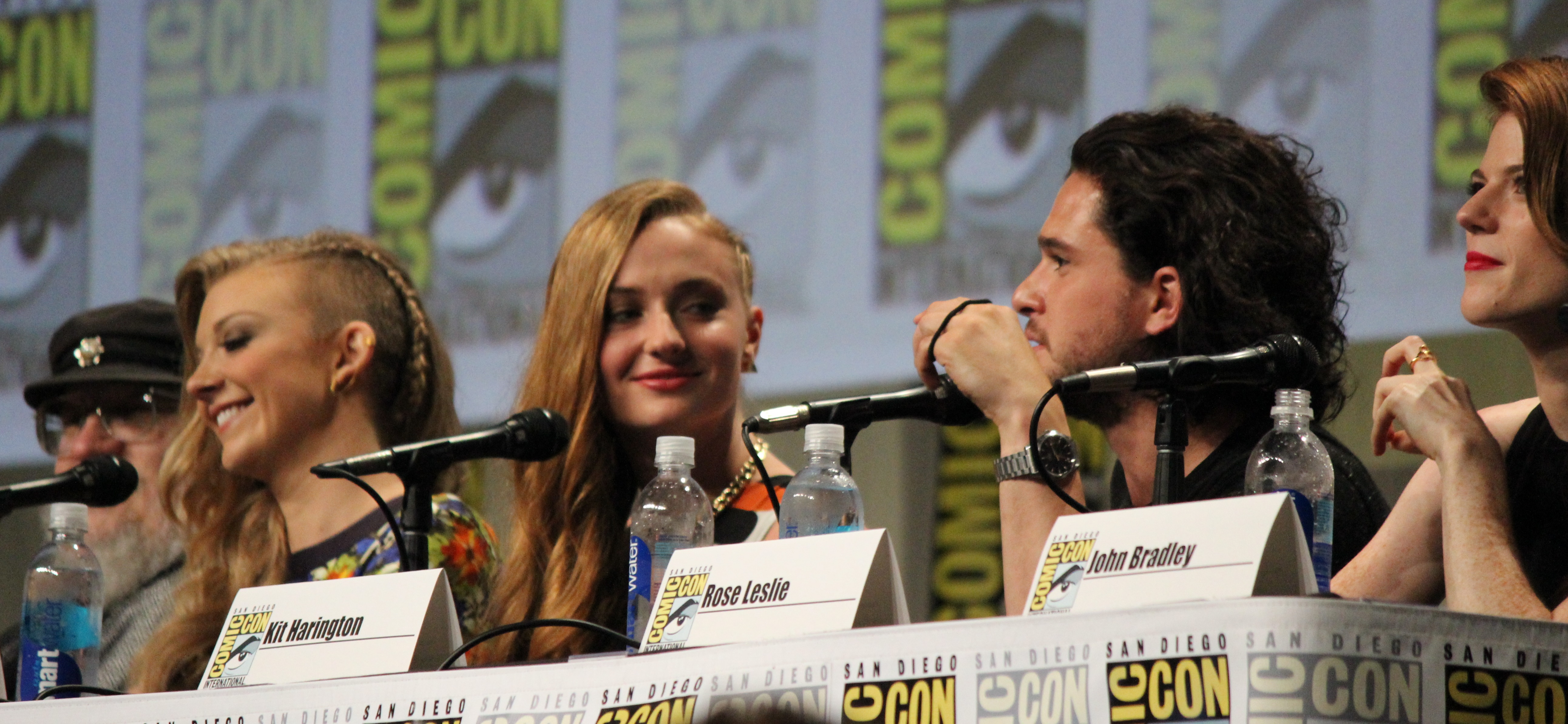The image depicts a panel at San Diego Comic-Con featuring members of the Game of Thrones cast. Seated behind a long table draped with a Comic-Con logo are five individuals, including John Bradley, Rose Leslie, and Kit Harington. Each cast member is seated in the center of the frame, visible from the shoulders up. Directly in front of each person is a nameplate and a microphone on a stand, with bottles of Smartwater placed next to them. The cast members exhibit a variety of features – pale skin, red, black, and blonde hair, a gray beard, and are dressed in diverse attires, such as a gray shirt, an orange, black, and white shirt, and a green, blue, white, and black shirt. The backdrop prominently displays the San Diego Comic-Con branding in white, yellow, and black, accented with a stylized eye logo. The setting captures the cast in mid-discussion, likely answering audience questions, fully immersing in the Comic-Con atmosphere.